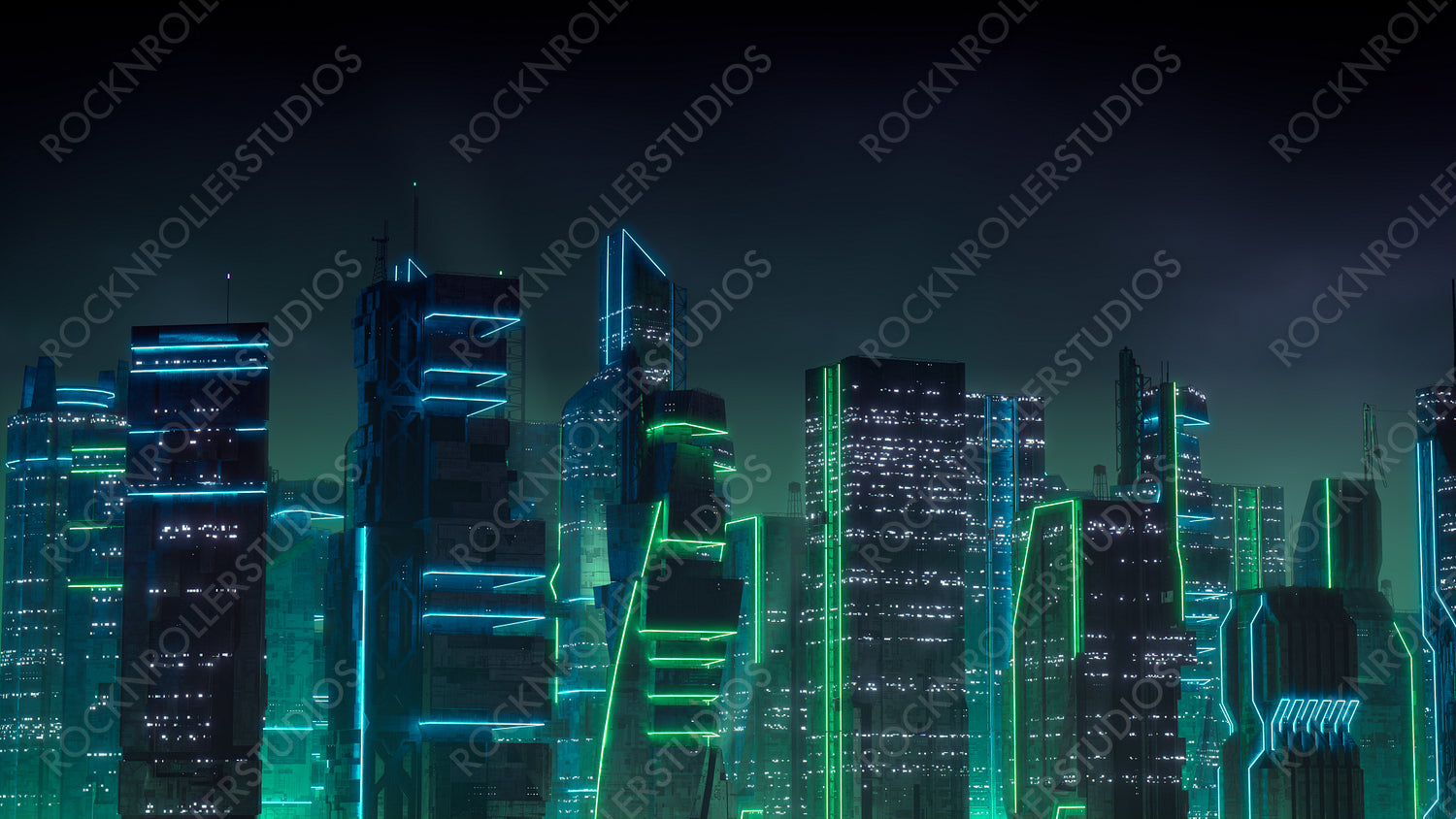A meticulously crafted image showcases a nighttime cityscape, dominated by a cluster of dark grey skyscrapers stretching against the night sky. The buildings are adorned with a multitude of horizontal lights, some glowing in shades of blue while others exude a pale green aura. Each skyscraper is punctuated with tiny lights on each floor, hinting at their multifaceted use as either office spaces or residential areas. Adding a touch of authenticity to the composition, the faint grey or white letters spelling out "Rock and Roll Studios" are diagonally superimposed across the background, unmistakably marking this shot as a product of studio ingenuity. The uniformity in height among the skyscrapers, coupled with the interplay of lights, creates a visually compelling urban panorama.